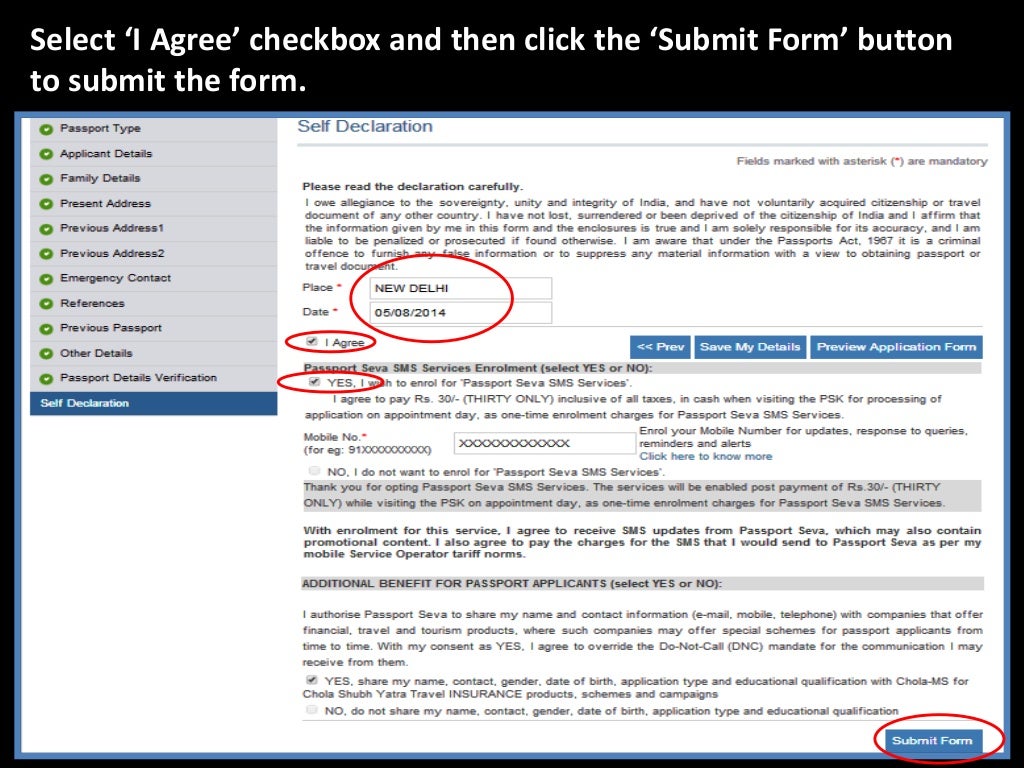---

**Caption for an Instructional Screenshot:**

The instructional screenshot features a form titled "Self-Declaration" against a black background with white text at the top. The text instructs users to select the "I agree" checkbox and then click the "Submit Form" button to submit the form. The image highlights key areas with red circles for clarity.

At the top of the form, the declaration states, "I owe allegiance to the sovereignty, unity, and integrity of India," followed by a detailed blurb. On the left side, a navigation bar with green check marks indicates the completed sections of the form, with this section being the final one.

Highlighted to the right of the blurb, the location "New Delhi" and the date "May 8th, 2014" are filled in specific fields. Below these fields, an "I agree" checkbox is checked, flanked by blue buttons to either go back or preview the application.

A separation bar below this section introduces another title. The next highlighted area includes the checkbox for "Yes, I wish to enroll for passport SMS services," circled in red. Additional blurbs provide further instructions, with options to enter a mobile number or select "No" if opting out of the service.

Further down, there are more detailed gray and black text blocks discussing authorization, followed by a yes or no checkbox. At the very bottom right corner, the "Submit Form" button is prominently circled in red, signaling the final step.

This comprehensive guide ensures clarity in completing and submitting the self-declaration form efficiently.